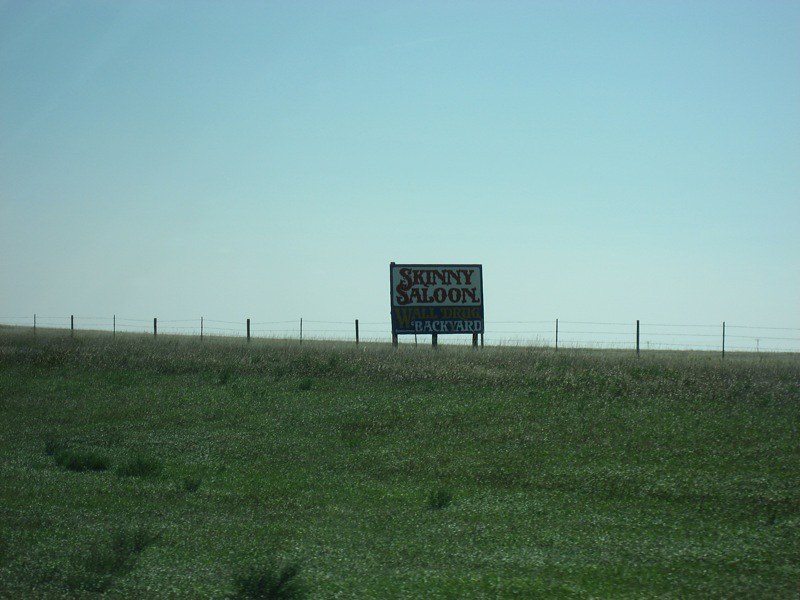This captivating landscape photograph features a lush, green field that extends roughly halfway up the frame. The horizon, marked by a nearly horizontal line that gently slopes upward to the left, demarcates the field from the sky. Just above this horizon runs a barbed wire fence, stretching across the entire width of the image. Centrally placed on the horizon is a prominent sign. This sign is white and green with vibrant red text that reads "Skinny Saloon." Below this, in yellow text, possibly depicting some additional detail, appears the word "Wall," followed by an unclear word. Additional white text reads "Backyard" at the bottom portion of the sign. The upper half of the photograph is dominated by a clear blue sky, which becomes slightly hazy near the border with the green field, contrasting beautifully with the lush landscape below.